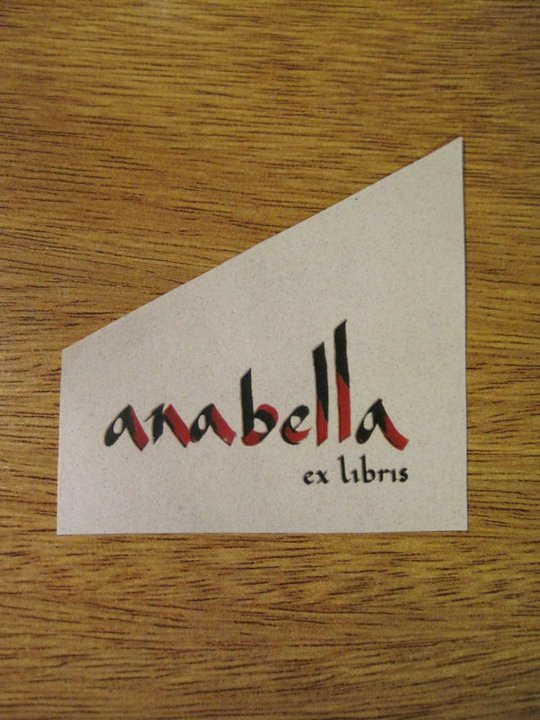The image depicts a small, uniquely shaped sign placed on a wooden surface with a medium-brown color and horizontally running dark brown grains. The sign, seemingly made of thick cardboard or light gray paper, has a distinctive trapezoidal shape featuring a low left side gradually rising to a sharp peak on the right. Centrally, the word "Annabella" is prominently displayed in a calligraphy style, combining black and deep red hues for a visually striking effect. Below "Annabella," in smaller, entirely black calligraphy, is the term "Ex Libris." The wooden surface, possibly a table or countertop, complements the sign's aesthetic with its natural, golden-brown tones.